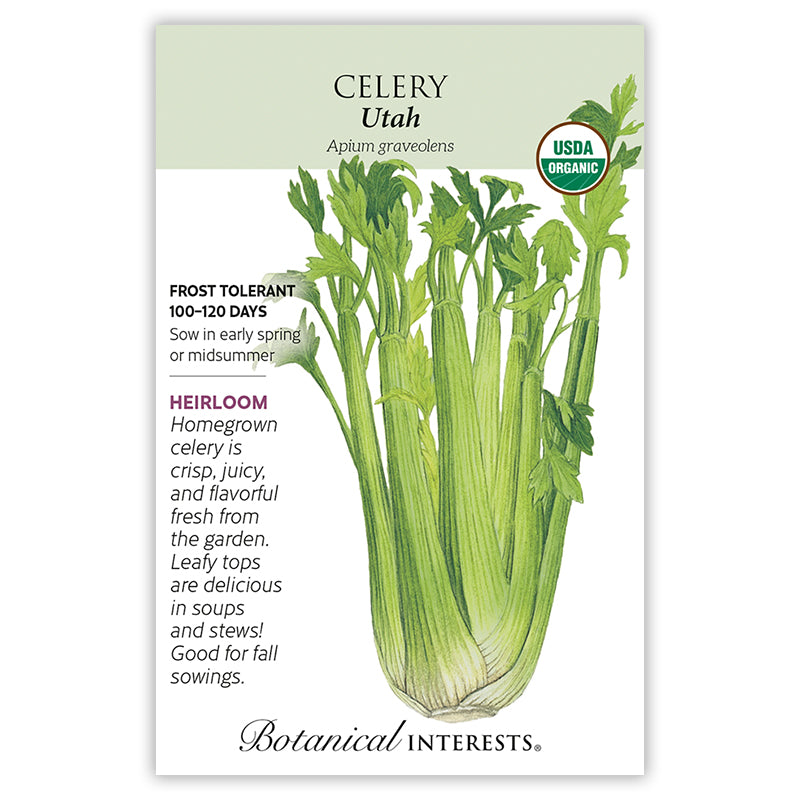The front of the seed pack features a detailed image of green celery with stalks and leafy tops grouped together. At the top, a light green background highlights the bold text "Celery, Utah" alongside its scientific name, Apium graveolens. The top right corner displays the USDA Organic logo, a brown circle with a white semicircle on top and a green semicircle on the bottom, marked with "USDA" in green and "organic" in white letters. To the left, black text provides information: "Frost tolerant, 100 to 120 days. Sow in early spring or midsummer." Below a red line, the word "heirloom" is emphasized in red or possibly purple text. Additional text in black reads, "Homegrown celery is crisp, juicy, and flavorful fresh from the garden. Leafy tops are delicious in soups and stews, good for fall sowings." At the bottom, the brand name "Botanical Interests" appears. The background of the pack is predominantly white, making the celery illustration and text stand out.